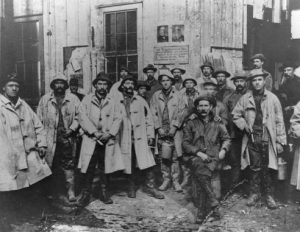This is a small, pixelated black-and-white photograph depicting a group of roughly 18 to 20 men in what appears to be an Old West scene. Central to the image, the men are wearing long, heavy coats, hats, and boots, with many sporting mustaches. The men seem to be posed for a picture, standing and one sitting on the trunk of a tree. They appear to be aged between 25 and 45 years old. In the background is a wooden building, possibly a sheriff's station or a bar, suggesting a late 1800s or early 1900s setting. The image quality is poor, making finer details and the text on the building's sign difficult to discern. Highlights on the top left corner of the photograph may indicate reflections of lights, implying that this is a photo of a print rather than a scan.